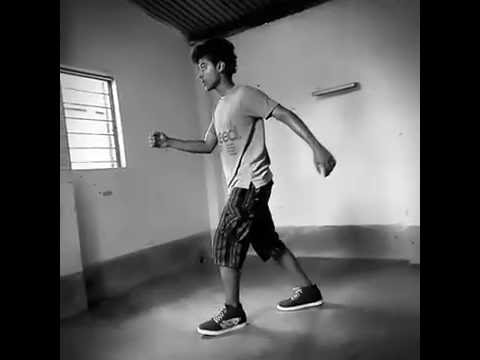The black-and-white photograph features a young man, seemingly in his 20s, captured mid-stride, facing towards the left in an empty room. He has short, thick dark hair and is wearing a light grey t-shirt with partially visible lettering, and long plaid shorts. His outfit is completed with black sneakers that have white soles and white laces. Positioned near the corner of two white walls, the room has a slightly slanted black ceiling and a grey floor. There is a rectangular window with six horizontal bars on the left wall and a handlebar or shelf mounted on the opposite wall. His arms are dynamically swung with the right arm extended in front and the left one behind him, while he steps forward with his left leg and leaves his right leg trailing. Two vertical black strips frame the sides of the photograph, adding an elegant edge to the composition.